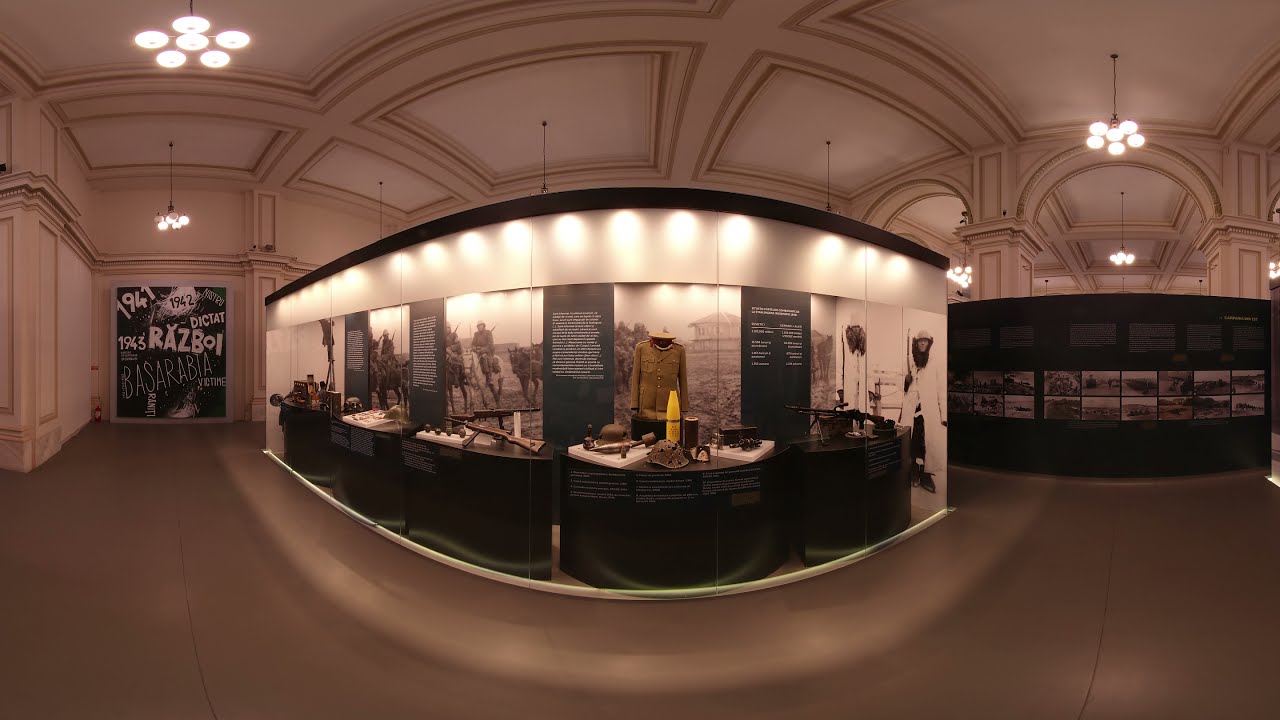The photograph captures a large, indoor exhibition space, featuring high beige walls and ceilings, estimated to be at least 10 to 15 feet tall. The center of the room is dominated by a war-themed display, showcasing various artifacts such as guns, uniforms, grenades, and a white-yellow missile. The display sits on black platforms, and nearby are two white army figures and horses in white and brown. The floor throughout the space is gray and hard. 

Illumination is provided by multiple white lights hanging from black wires, with the ceiling trimmed in brown or gold. In the backdrop, there is text on a sign that reads “1941” in white, “1942” in black on a white background, “Dictate” in white, “Rays,” “Rasboy” in white, “1943” in white on a black background, and “Basarabia.” Although numerous description boards and an array of pictures surround the exhibit, the text is not legible. The overall color palette includes shades of tan, yellow, green, brown, black, and white, suggesting the setting is likely a meticulously curated army museum.